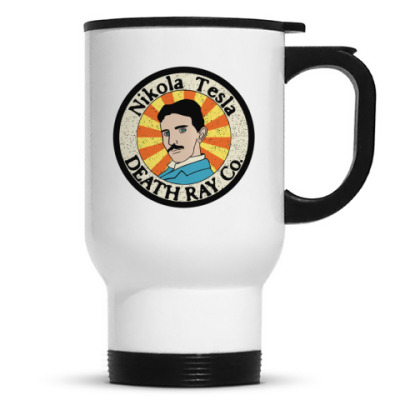This color photograph is a detailed product image of a tall, white travel coffee mug, commonly used for promotional or retail purposes. The mug, likely made of plastic or coated metal, is positioned against a bright white background, resembling a white light box setup. It features a sleek design tapering down to a narrower black base and has a black lid at the top. A black handle extends to the right, creating a balanced visual with its black accentuations at the top and bottom.

Central to the mug's design is an eye-catching graphic prominently displayed on the front. This graphic consists of a circular logo with dual concentric circles. The outer circle contains the text "Nikola Tesla" in black serif font at the top and "DEATH RAY CO." in black, all capital letters at the bottom. Inside this external circle is another smaller circle that showcases radiating orange and yellow segments, simulating sun rays. Superimposed over these radiating segments is a cartoon depiction of Nikola Tesla. He is illustrated with short, dark brown hair and a thin mustache. Tesla is depicted looking over his left shoulder, dressed in a light blue jacket and a white shirt, making the graphic both vivid and memorable.

Subtle shadowing at the base of the mug enhances the realism of the image, grounding the product against its pristine backdrop. This meticulous portrayal underscores the style of photographic representationalism and product photography, highlighting both aesthetic and functional design elements.